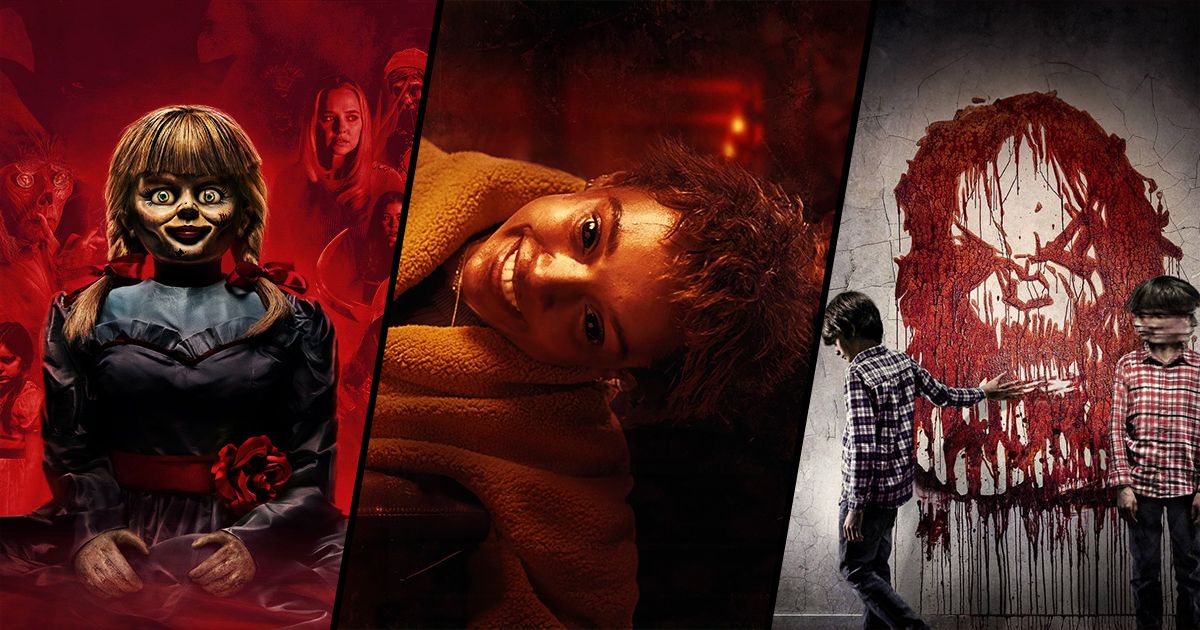The image is a full-color, wide promotional display featuring three distinct horror movie posters. On the far left, the poster for "Annabelle" showcases an eerie, old-fashioned child's doll with dark brown hair styled in pigtails tied with red bows, and dead eyes gazing forward. The doll wears a black dress accented with a red belt. Behind it, a blood-red background reveals shadowy figures and possibly a demon, adding to the sinister atmosphere. 

The middle poster presents a young Black woman clad in a yellowish-brown robe. She is leaning sideways, almost hanging off a table or couch, with her eyes unnaturally wide and entirely black, paired with a disturbingly large grin that exudes an evil presence.

On the far right, the poster believed to be for "Sinister" depicts two young boys in front of a white wall. One boy is seen dragging his hand through a crimson drawing of a demonic face, with blood dripping down the wall. The other boy appears to be morphing, his head blending through different phases, creating an unsettling, multi-faced image.

Overall, the promotional display effectively captures the terrifying essence of each movie through vivid and grotesque imagery.